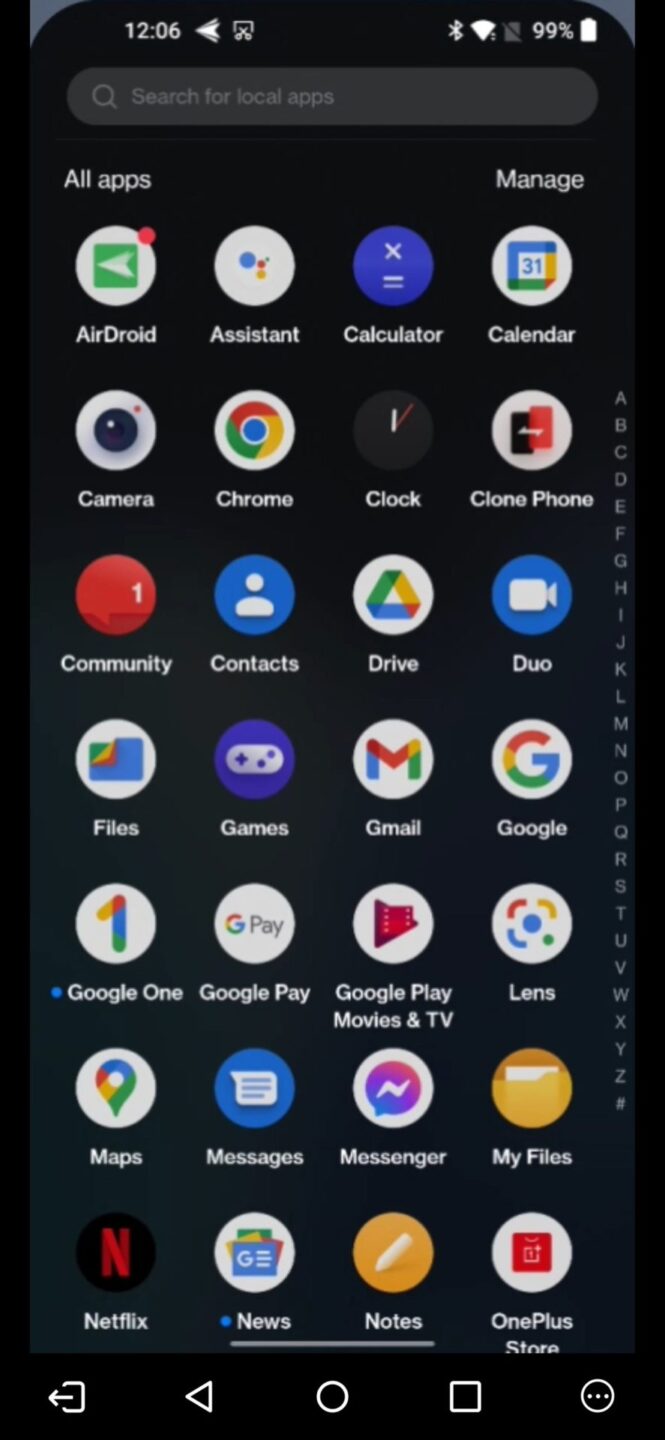This image depicts the apps section of a OnePlus mobile device, showcasing a neatly organized interface in dark mode. The background is black, indicating the user has enabled the dark theme.

At the very top of the screen, the status bar displays the time as 12:06 on the upper left. Adjacent to the time, icons are present for various statuses: a white airplane or paper plane symbol, a clip symbol, Bluetooth, Wi-Fi, cellular signal strength, and battery life at 99%.

Beneath the status bar is a search bar for locating local apps swiftly. The main section of the screen showcases the app grid, formatted into seven rows with four apps per row. The app icons are:

1. **First row**: AirDroid, Assistant, Calculator, Calendar
2. **Second row**: Camera, Chrome, Clock, Clock
3. **Third row**: Phone, Clone Phone, Community, Contacts
4. **Fourth row**: Drive, Duo, Files, Games
5. **Fifth row**: Gmail, Google, Google One, Google Play
6. **Sixth row**: Google Play Movies & TV, Google Lens, Maps, Messages
7. **Seventh row**: Messenger, My Files, Netflix, Google News, Notes, OnePlus Store

At the bottom of the screen, there are the standard Android navigation buttons: Back, Home, and Tabs.

Overall, the image provides a clear view of the OnePlus device’s app organization, user interface, and the utilization of dark mode to reduce eye strain.